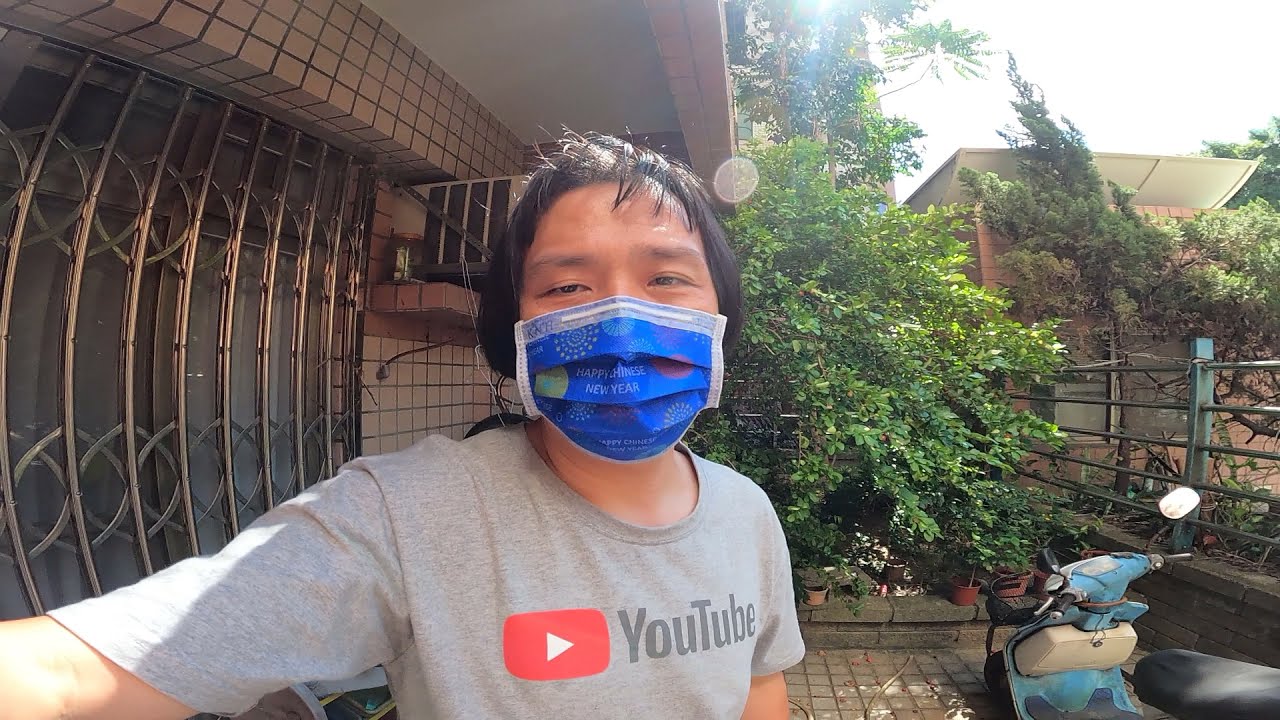The image captures a person with short dark hair and brown eyes, appearing to be of Asian descent, taking a selfie while looking directly at the camera. They are wearing a blue facial mask and a gray t-shirt featuring the YouTube logo, which includes a red rectangular play button icon. The setting is outdoors on a bright, sunny day. To the right of the person is a blue and white moped, with green shrubs and trees, a wooden fence, and part of a house visible behind it. To the left, there appears to be a storefront or a building with curved metal bars and tiled surfaces, and a checkered background that adds to the colorful composition of the scene. The ground is a brick-like tile, and sunlight is peeking through the trees, enhancing the overall brightness and vividness of the photo.